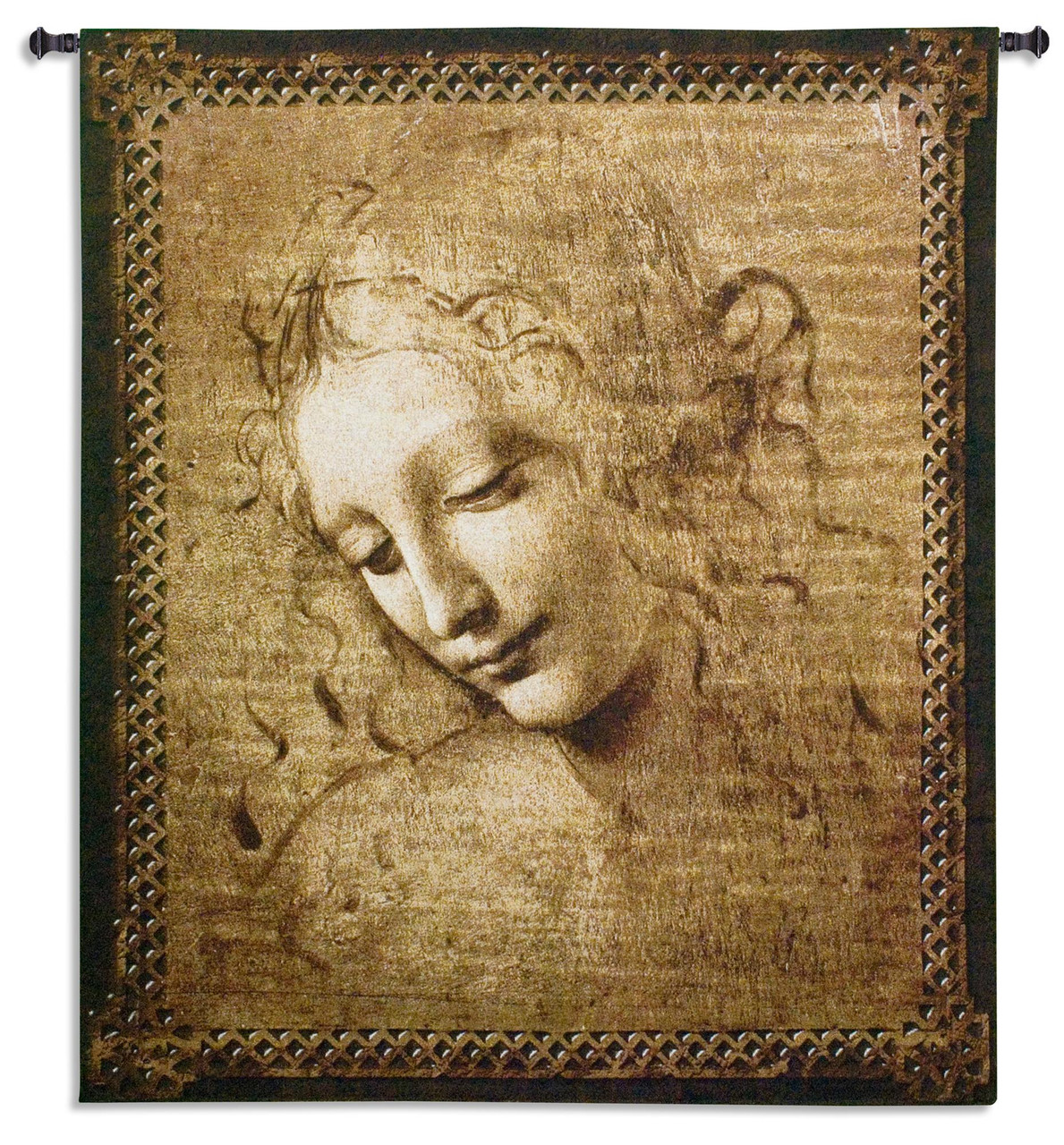The image depicts an antique-looking drawing, resembling a piece of wall art hanging from a black metal rod with bulbous ends, much like a shower rod, with its two ends visible at the top left and right. The artwork itself features a dark, possibly black, background and is either on rusted steel or aged fabric, giving it an ancient, well-worn appearance. Surrounding the drawing is a border consisting of small diamond shapes, adding a distinctive embellishment to the piece. The central figure is a young woman with loosely curled hair cascading around her face. Her head is tilted slightly to the left and downward, her eyes partially closed, almost in a contemplative or serene expression. She displays soft facial features, and a hint of a smile can be seen on her lips. The overall effect is that of an old, intricate tapestry or banner, bringing a touch of vintage elegance to the artwork.